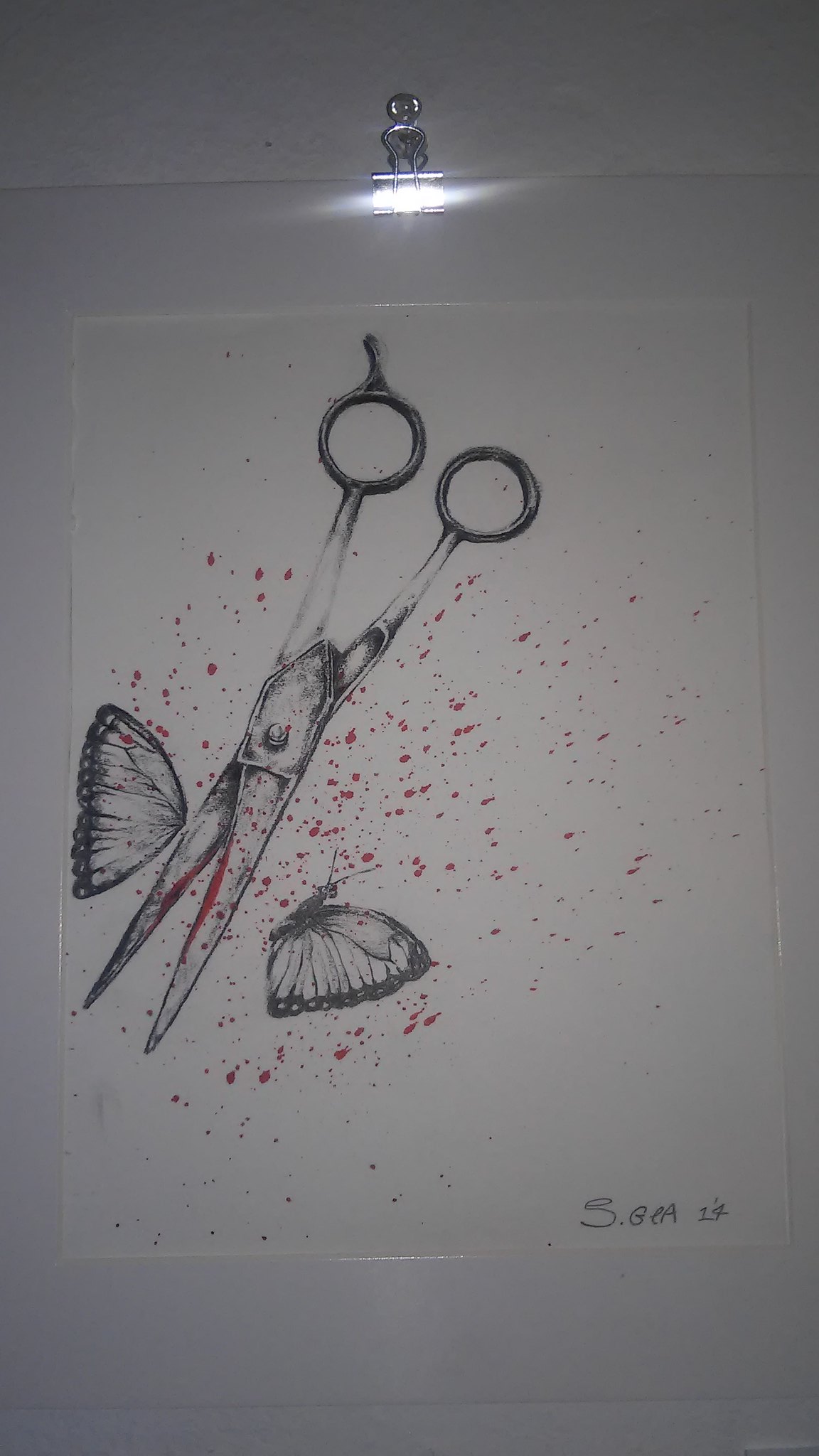The artwork is a vertical print presenting a haunting portrayal of a pair of scissors cutting a butterfly in half. The composition is set against a muted gray background. The image is supported by a metallic binder clip attached to a hook on the wall, displaying the print matted but unframed. The white matting surrounds the central image, which could either be a detailed print or intricate drawing. 

The disturbing focal point is a pair of long, sharp scissors depicted upside down, positioned from the top to the bottom of the artwork, slightly opened. A small knob protrudes from the left blade. The scissors' blades are stained with splattered blood, contributing to the macabre atmosphere. The butterfly, split in half by the scissors, has its two separate wings on either side of the sharp blades, hinting at the brutality of the act.

In the lower right-hand corner, the artist has signed their initials along with a year that appears to be either '14 or '17, adding a personal touch to the provocative piece.